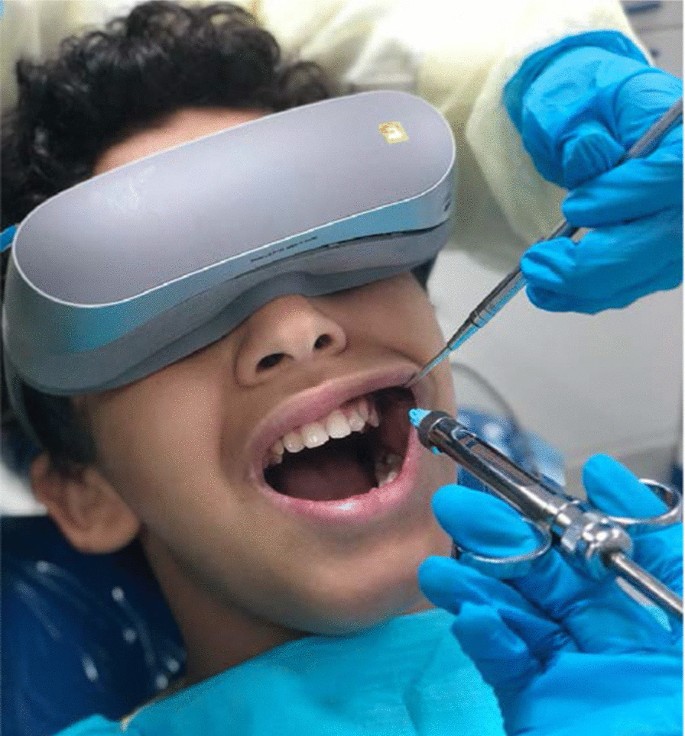This image captures a moment in a dental procedure involving a young boy with dark black curly hair, who appears to be a teenager at most. The boy is seated in a dentist's chair, his mouth wide open, likely held open for treatment. He is wearing flat, gray virtual reality goggles, presumably to keep him entertained during the procedure. 

In the upper part of the image, a medical professional wearing a white gown and blue rubber gloves on their left hand is visible. This person is holding a dental tool that helps keep the boy's mouth open. From the lower right of the image, another blue-gloved hand, possibly from a different dental assistant, is poised with a silver instrument that might be a needle poised for injection, possibly as part of a numbing process. The dentist appears to be standing behind the boy, meticulously coordinating the procedure.